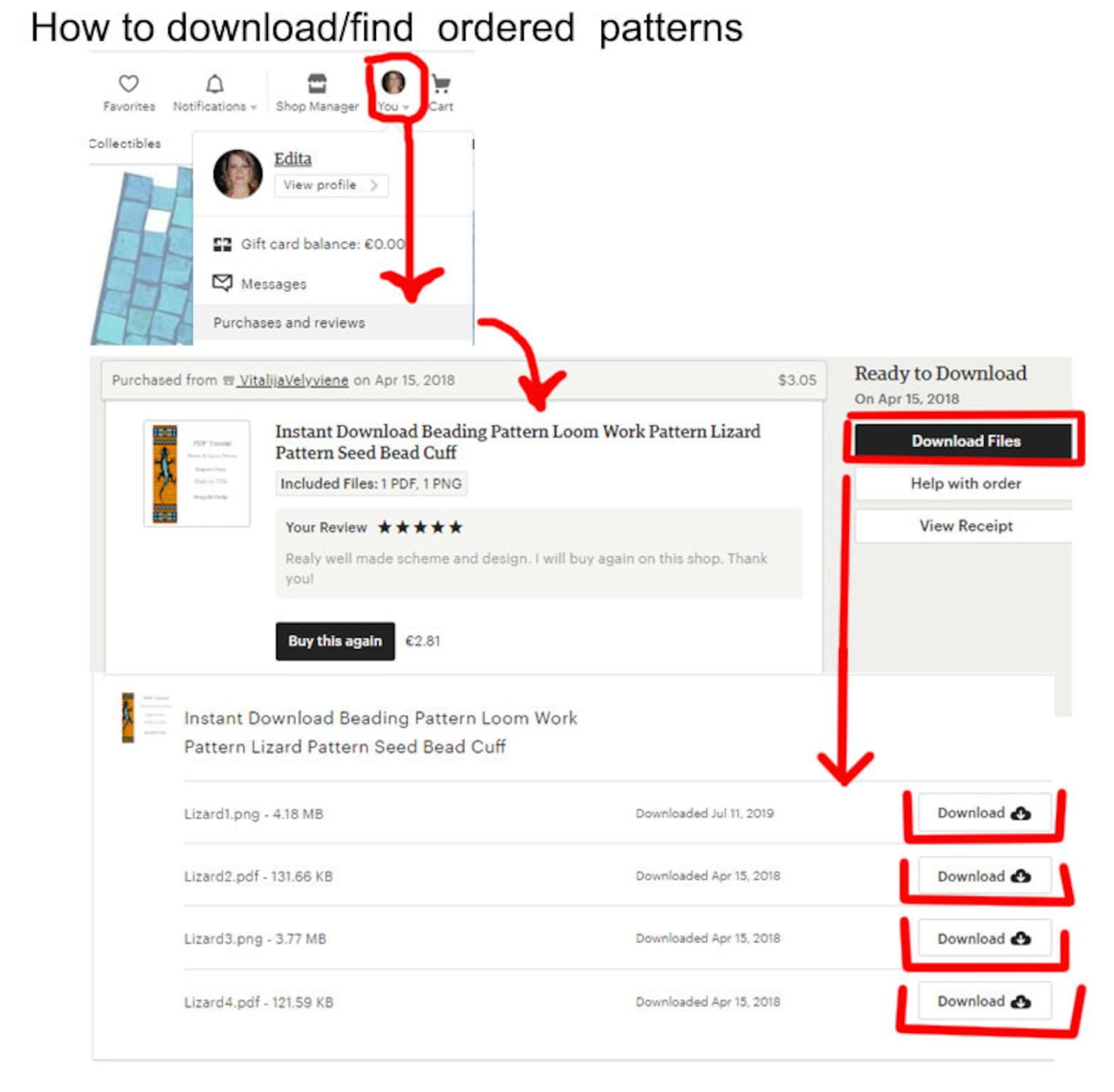This webpage demonstrates how to download ordered patterns. The title, "How to Download Find Ordered Patterns," is prominently displayed at the top. Below this, a screenshot of a user's profile is shown, featuring highlighted tabs labeled Favorites, Notifications, Shop Manager, You, and Cart Collectibles. 

The "You" tab is emphasized with a red paint tool, accompanied by a downward-pointing red arrow and another arrow pointing to the right and downward. This leads to a section titled "Purchase from a Company," which displays a pattern named "Instant Download Beading Pattern: Loom Work Pattern - Lizard Pattern - Seed Bead Cuff." A star rating and a handwritten review of the product are visible, along with a "Buy this item again" option.

Adjacent to this information is a section labeled "Ready to Download," enclosed in a red rectangle with a downward-pointing red arrow. Below, options like "Help with Order" and "View Receipt" are available. The "Instant Download Beading Pattern: Loom Work" section reappears, listing four PNG files ready for download. Each download tab next to these files is highlighted in red.